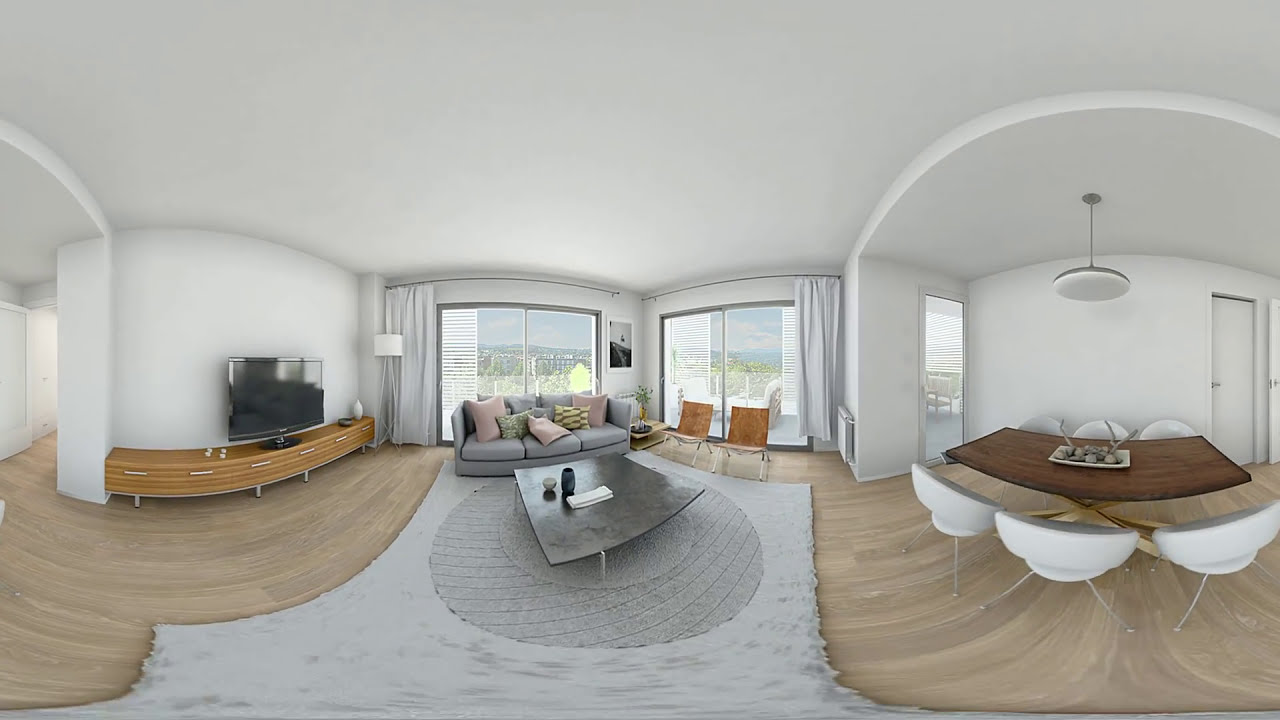This image showcases a panoramic view of a modern, white living room, reminiscent of a chic Miami condo. The walls are pristine white, accented by several striking archways. The flooring appears to be a light tan or beige hardwood, harmonizing with the room's light, airy feel. Centrally placed upon the flooring is a uniquely shaped gray carpet, atop which sits a stylish gray rock slab coffee table, adorned with various objects.

A low, modernist wooden TV stand housing a black television set is situated on the left side of the room. The stand, much like other pieces of furniture, is constructed from light wood, contributing to the minimalist aesthetic. Adjacent to the TV stand is a white bar that descends in an arch and intersects with another white panel.

In the heart of the living room, directly centered in the image, stands a light gray couch with plush pillows. Flanking it are two brown chairs, and collectively these seating elements face the distinctive coffee table. Large windows, draped with sleek white curtains, offer a panoramic view that suggests a vibrant cityscape, possibly Miami.

Further to the right, another expansive white arch encapsulates a modern dining area. This area features a rectangular, curved brown table paired with white, contemporary chairs. The room is well-lit, indicating that the photo was taken during the day. This inviting, elegant space is clearly designed with both aesthetics and comfort in mind.